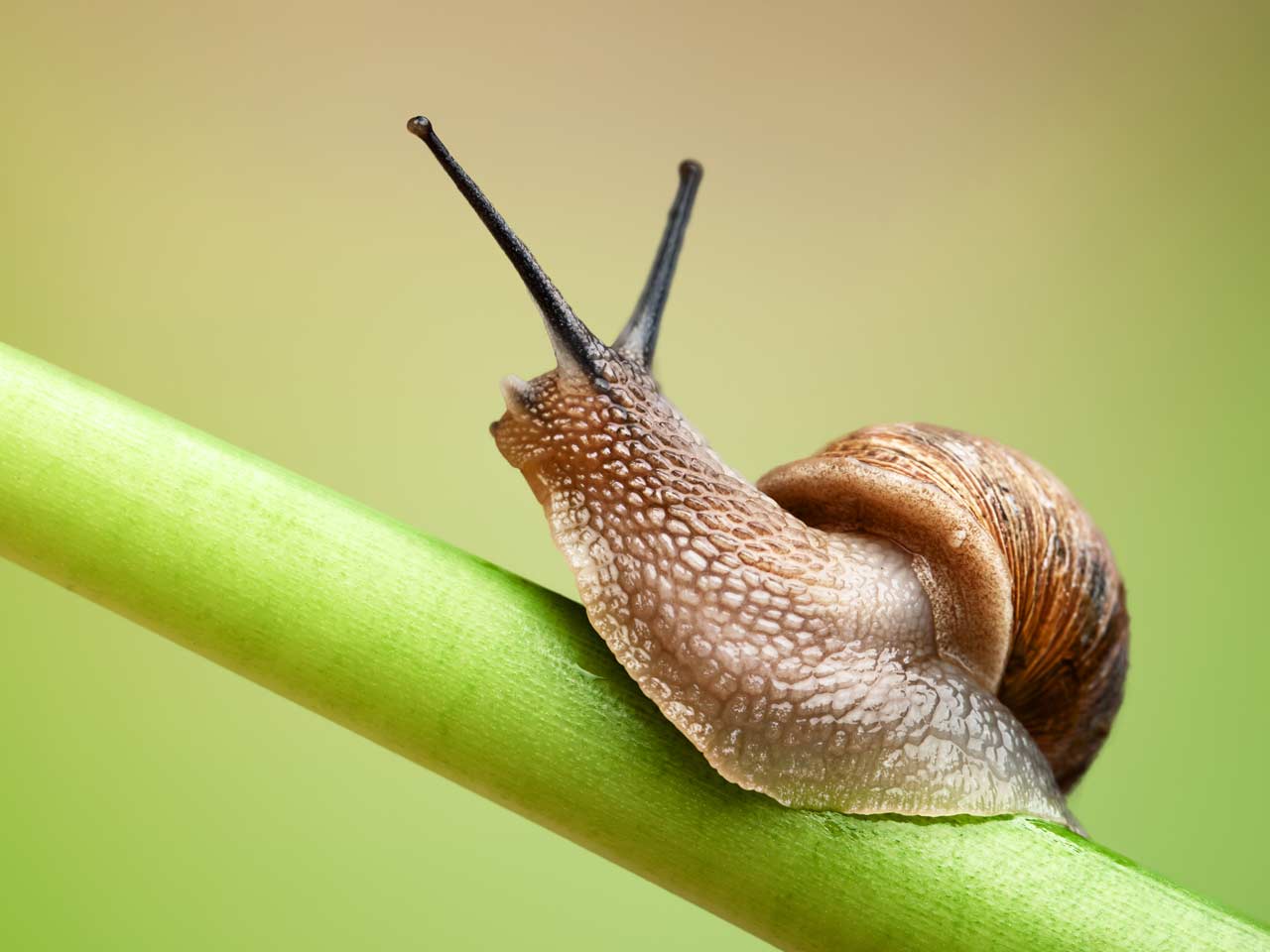The image captures a zoomed-in, detailed view of a brown snail with a dark brown, lighter brown, and white body, crawling on a vibrant green stalk in an outdoor setting. The snail's rough, slimy skin is visible, with its black antennae extending left and right. The left eye bulge is discernible. The shell, also brown with black and white accents, exhibits striations. The background is heavily blurred with green, white, and yellow hues, giving the impression of a bright, sunny day. The snail is heading upwards, with a focused, purposeful demeanor. The overall composition of the image is in a square format, emphasizing the intricate details of the snail and its movement on the plant stalk.